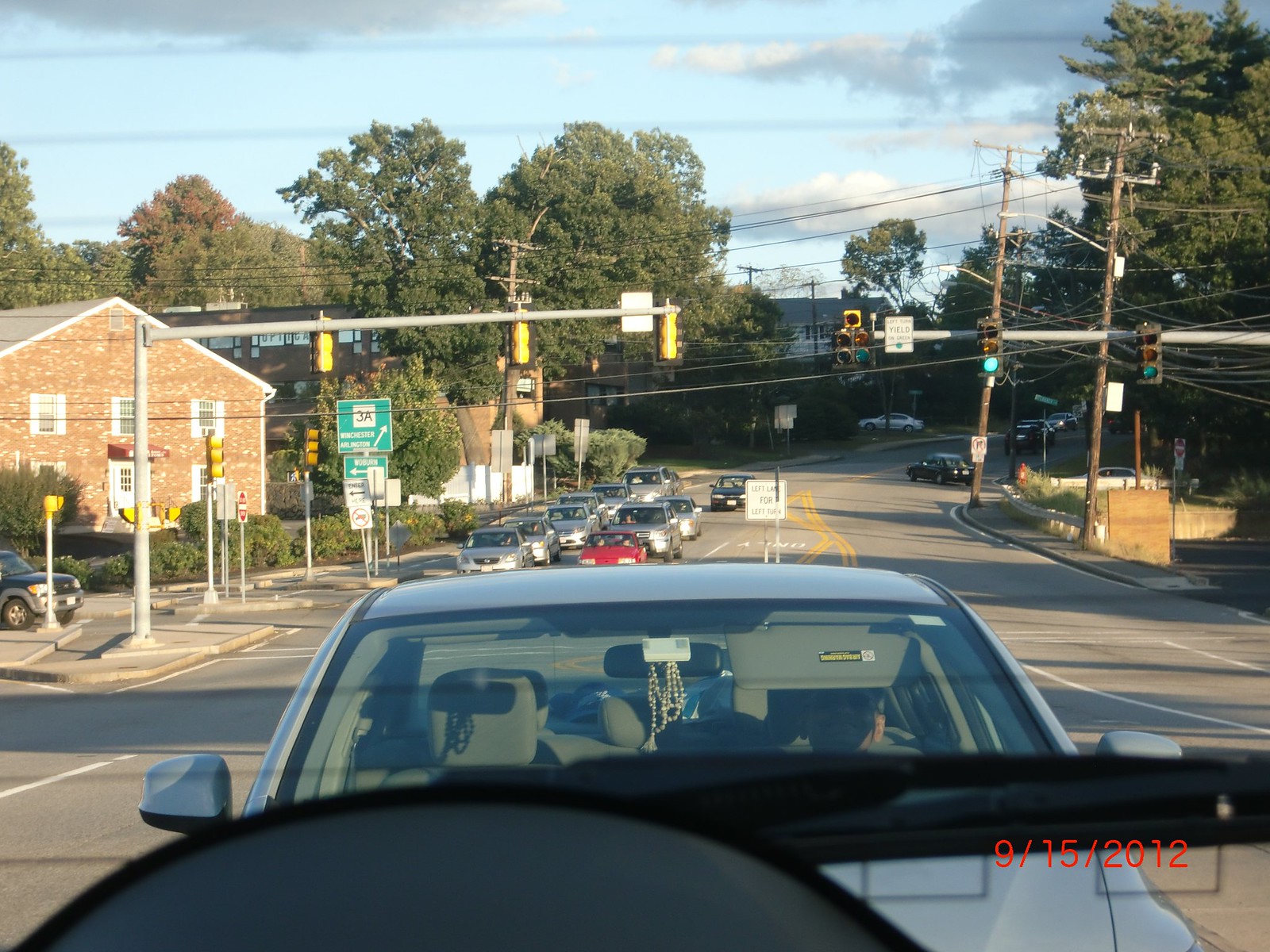This image, dated 9-15-2012 as indicated by red text in the bottom right corner, is taken from inside a car, likely through a dashcam on the driver's side. The composition captures a sprawling scene through the windshield. Above, the sky is blue with interspersed clouds, and electrical lines stretch across the top, supported by telephone poles scattered throughout the midsection of the image. The foreground shows a gray road with yellow lane markings near the bottom. Multiple cars are visible: one particularly close, tinted a bluish-gray, appears directly ahead, while several others are stopped around 10-20 meters back at a traffic light junction, where the light is green. To the left, farther back, a line of cars waits at the intersection. There is a brick house and a green sign with '3A' in white text towards the left side of the image. Within the car itself, parts of the dashboard, including a sun cover, and an object, possibly beads, hang from the rearview mirror. The atmosphere hints at an everyday moment captured on a road trip or commute, with structures, vehicles, and vivid details blending into an encompassing scene.